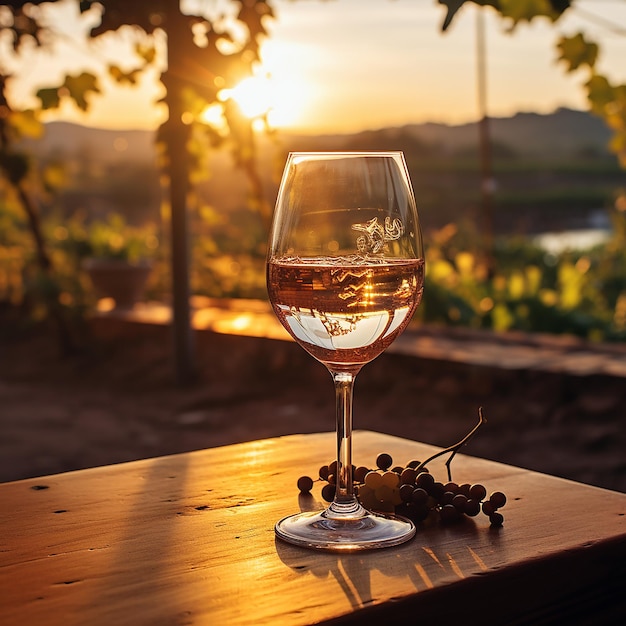The image captures a rustic outdoor scene featuring a clear, stemmed wine glass half-filled with what appears to be white or rosé wine, placed slightly right of center on a light brown wooden table. The glass has a round, stable base and appears to have some engraving on its front side, adding a touch of elegance. Surrounding the glass on the table are clusters of white and red grapes, and a few darker berries or cherries with stems, adding a natural touch to the composition.

In the background, the image shows an unfocused yet scenic vista with a mix of greenery, including trees and a possible grassy area, and farther into the distance, hills or mountains. The serene sky above these hills suggests that the photo was taken in the late afternoon, with the sun either setting or rising, casting a golden hue over the scene. A small ledge or wall runs across the upper part of the photo, and there might be a hint of a lake, enhancing the tranquil ambiance. The overall setting exudes a rustic, peaceful charm, with the focus keenly on the wine glass and grapes in the foreground.